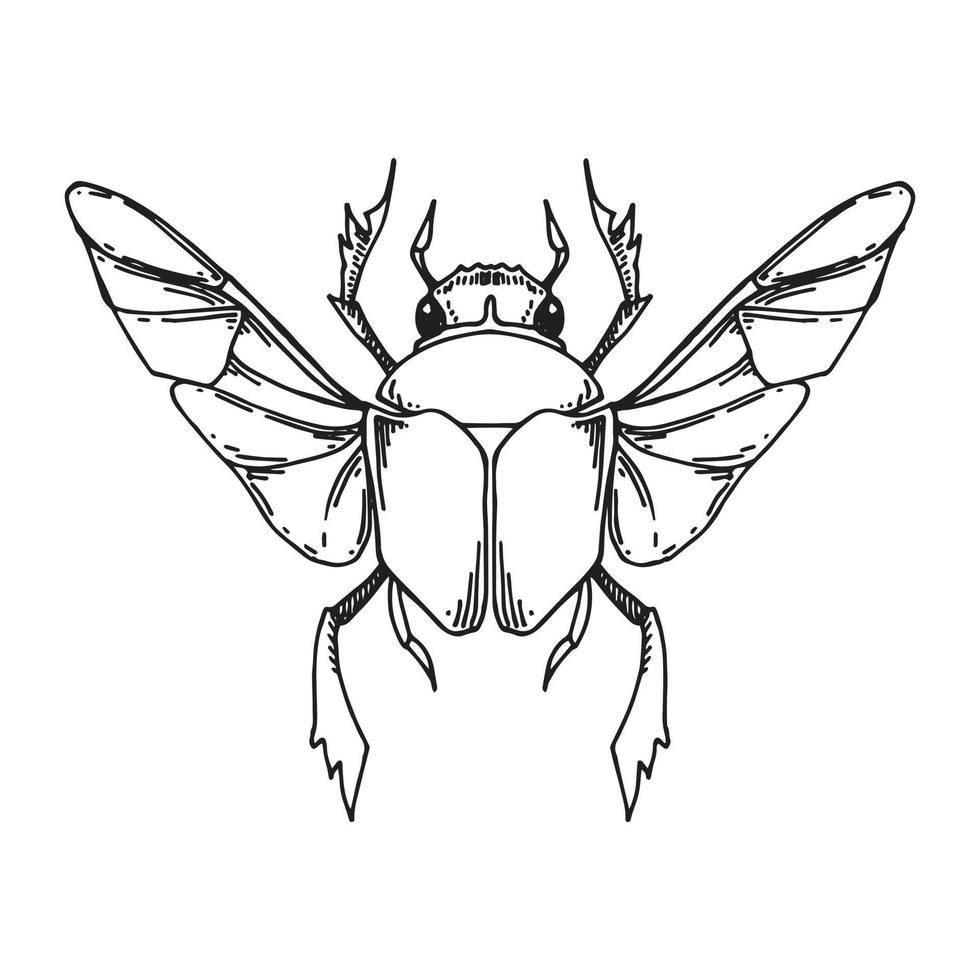The image features a detailed black outline of a beetle-like insect set against a plain white background, resembling a drawing that could easily be colored in. The insect boasts a large, oval-shaped body that is intricately detailed with numerous lines, especially noticeable on its arms and legs. It has two prominent wings extending from either side, each sectioned distinctly, enhancing the intricate appearance. The beetle's anatomy includes two large eyes and two small pincers situated at the front. Additionally, it has two longer legs and two shorter legs positioned towards the rear and two more arms extending from the front. The detailed nature of the wings and limbs suggests that the insect appears capable of flight, with its specific features making it stand out prominently.